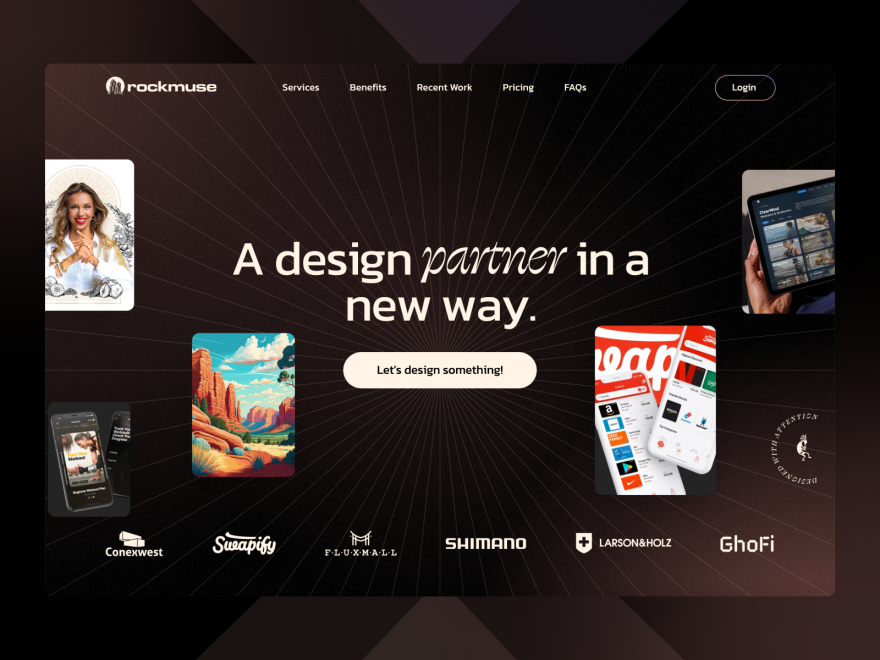The image features a sleek black box with a small white circle, in which a tiny black rock is depicted. Prominent text reads "Rock Muse" alongside navigation options: "Services, Benefits, Recent Work, Pricing, and Facts." There is a prominent black login button. 

On the left side, there is a picture of an attractive woman dressed in a light blue outfit. Above her, the text states, "A design partner in a new way," and nearby, a small white box reads, "Let's design something."

Towards the lower left, there's a phone displaying a vibrant image, surrounded by a picturesque scene of imposing rocky mountains, a clear blue sky with fluffy white clouds, a winding road, and various plants.

In the upper right corner, a person holds a screen showcasing multiple images, including beach scenes. Below, two phones display different menu interfaces. In the lower right corner, a semi-circle encloses an icon of a person with a backpack.

At the bottom, the names "Conic West, Swapify, Flumo, Shimano, Larson, Holtz, and Gophy" are listed in bold.